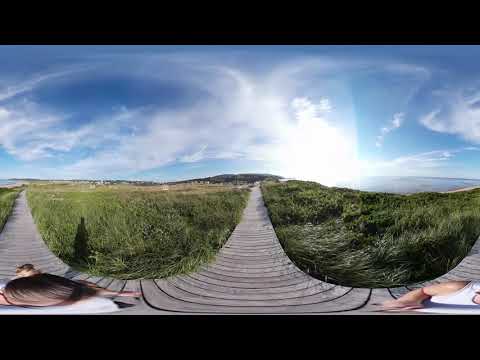The image features a panoramic view with black borders on both the top and bottom. The photograph captures a bright, sunny day with a blue sky scattered with white clouds. On the horizon, beneath the sky, gentle hills can be seen. In the foreground, the lower half of the picture appears distorted. 

A grayish wooden boardwalk spans the image, flanked by grassy areas that seem to form bowl-like depressions on either side of the walkway. The grass is tall, thick, and varies from dark to medium green, suggesting a marshy landscape. The boardwalk itself appears slightly warped, indicative of a panoramic shot.

Towards the lower left corner of the image, there's a stretched and distorted figure that resembles a bird, while the bottom right corner shows what appears to be a person, also distorted. Two individuals, each wearing white t-shirts and dark-colored pants or shorts, are visible on the left and right parts of the image, potentially taking pictures or using a selfie camera. The sun is positioned near the horizon on the right, indicating that the picture was taken either in the early morning or late afternoon.